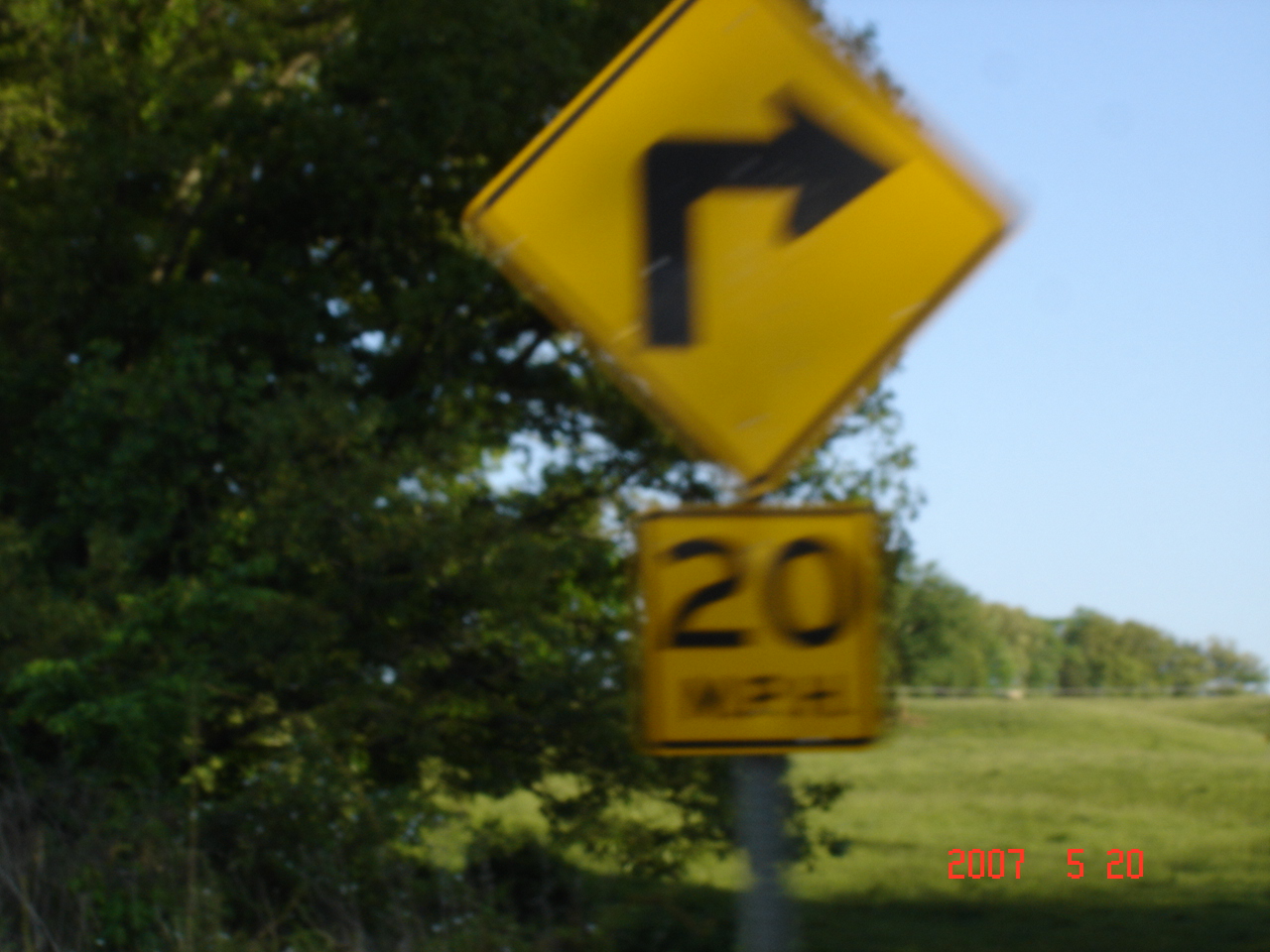This outdoor landscape photograph, taken on May 20, 2007, features a rectangular frame captured in a landscape orientation. The image is noticeably blurry, obscuring some of the finer details. At the forefront, there is a yellow diamond-shaped road sign with a bent arrow, indicating a curve, and directly below it, a square yellow sign with black lettering that reads "20 miles per hour," though the text is difficult to decipher due to the blur. Behind the sign stands a dark, shadowy tree, which casts shade over the immediate area, contrasting with the light blue, sunny sky above. Further into the background, a grassy meadow and a fence are visible, lining the boundary with additional trees beyond. The shaded foreground hints at the presence of another tree not visible in the frame, adding depth to the scene.